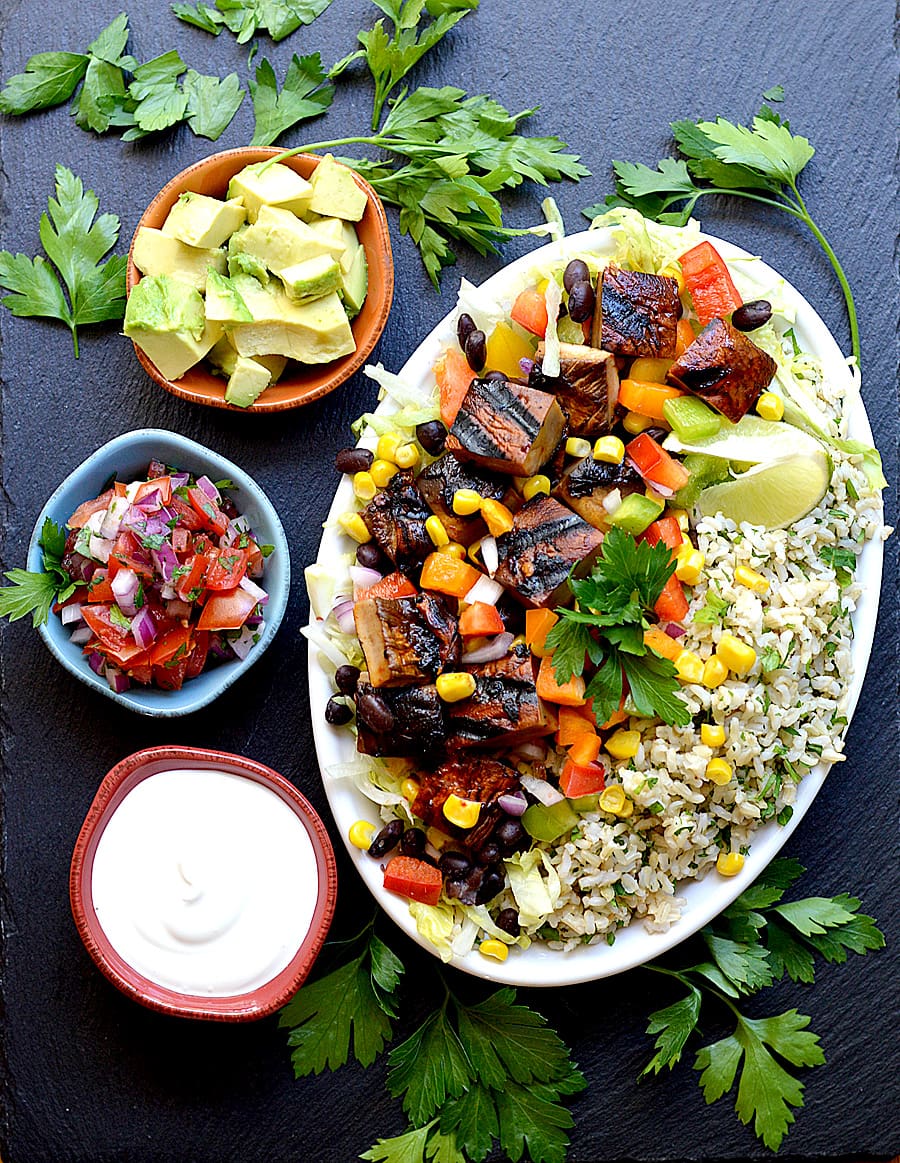This image presents an overhead view of a dining setup featuring a main plate on the right-hand side and three smaller dishes arrayed around it. The main plate, dominating the composition, serves as the centerpiece, housing the primary course. Surrounding this primary dish, three smaller bowls each contain distinct types of food. 

- The bowl at the top holds cube-shaped pieces of fruit, adding a colorful and refreshing element to the spread.
- The bowl positioned at the center left is filled with a vibrant mix of chopped tomatoes and onions, likely a fresh salad or a salsa.
- The bowl at the lower left contains a white, creamy substance, which might be a dip or sauce, perhaps made of yogurt or sour cream.

Adding to the visual appeal, sprigs of fresh parsley are artfully scattered across the table, bringing a touch of green and framing the plates in a natural, leafy setting. This thoughtfully arranged tableau invites the viewer to savor the variety of tastes and textures on offer.